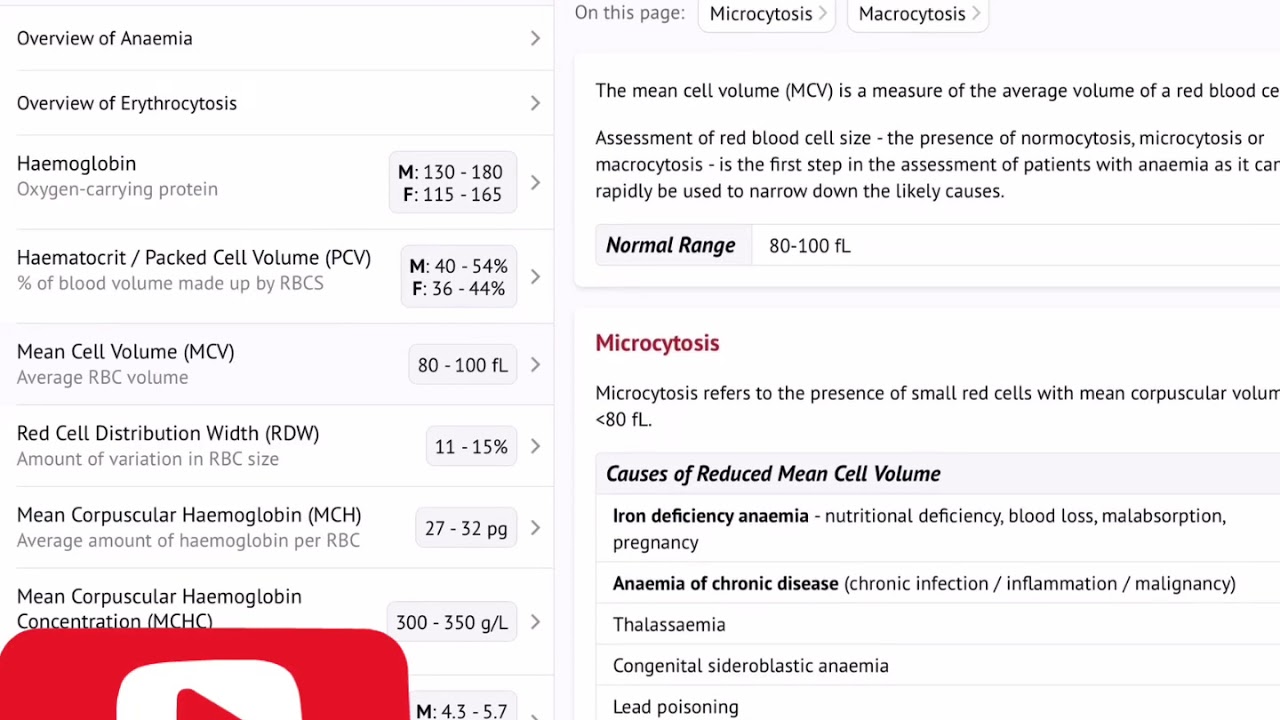The webpage displays a detailed medical chart or analysis focused on blood-related conditions. On the left side of the page, headings include "Overview of Anemia" and "Overview of Urocytosis," followed by numerical ranges and descriptions for various blood parameters such as Hemoglobin, Hematocrit, Mean Cell Volume, Red Cell Distribution Width, Mean Corpuscular Hemoglobin, and Mean Corpuscular Hemoglobin Concentration. To the right of these menu options, information is presented on Mycotosis and Macrotosis, each accompanied by its respective normal range and descriptions. The webpage features a stark white background with black text for clarity and a partially visible red play button located at the bottom left corner of the screen.